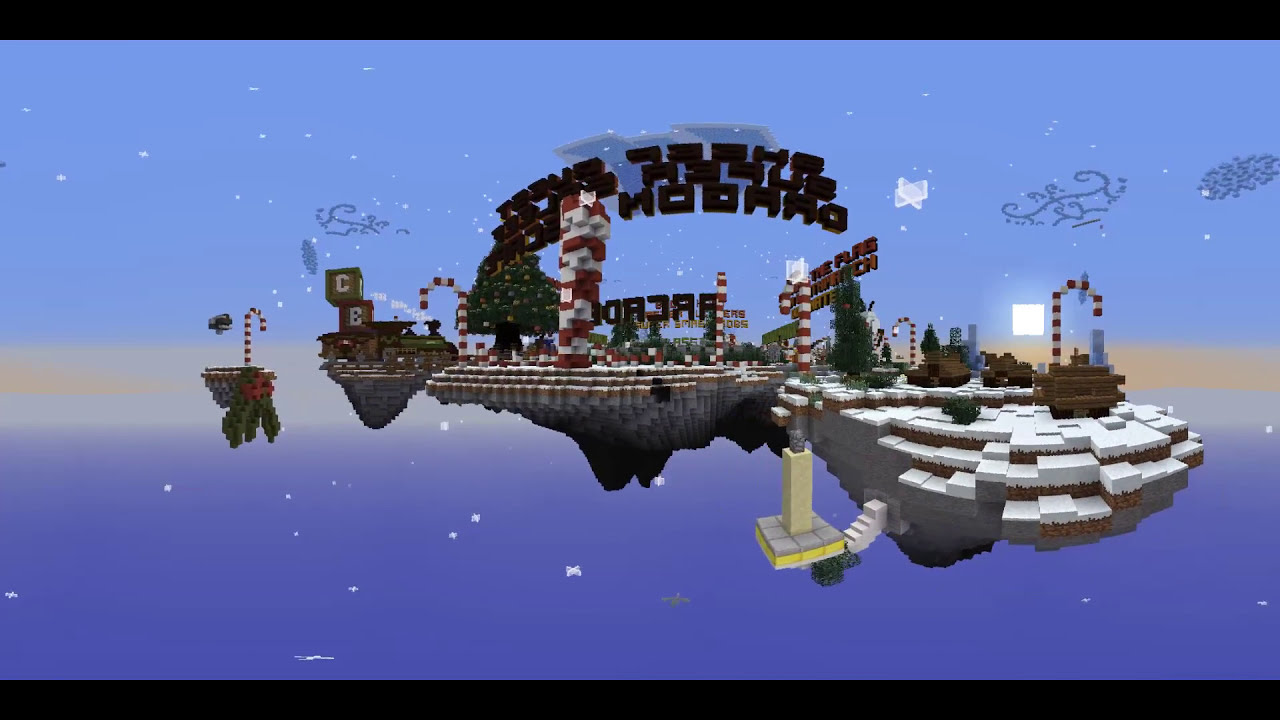The image depicts a festive, digitized 3D world that appears reminiscent of Minecraft but also draws comparisons to a Fortnite map or a Lego world. The floating landscape, set against a blue, starry sky, features various components that enhance its holiday theme. Prominent in the scene are several Christmas trees adorned with ornaments and colorful candy canes. There are also wooden toy blocks marked with the letters "C" and "E," and the overall design includes red, white, and green elements. The landscape includes multiple floating islands, with pine trees and presents scattered throughout. Additionally, there are some unreadable words at the top of the image that appear flipped backwards, contributing to the surreal, digitized appearance of this festive, floating creation.